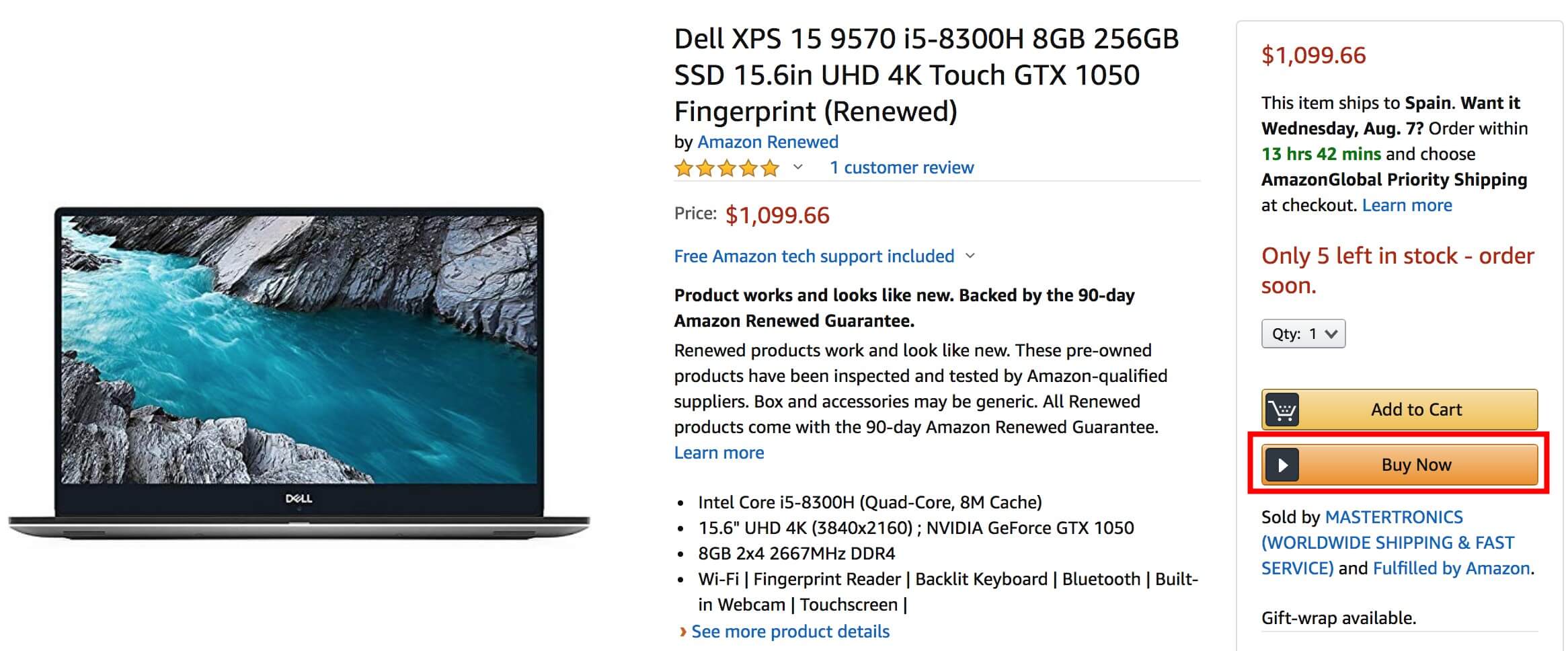The featured image showcases a Dell XPS 15 9570 laptop available for sale on a website, specifically Amazon. On the left-hand side of the page, there's a picture of the laptop. The base of the laptop is silver, and it features a black frame around the screen, which displays a serene scene of water flowing through rocks. The Dell logo is prominently displayed at the bottom of the monitor.

Next to the image, the product description is clearly outlined in bold black letters, reading: "Dell XPS 15 9570, i5-8300H, 8GB RAM, 256GB SSD, 15.6 inches, UHD 4K Touch, GTX 1050, Fingerprint Reader (Renewed)." This information indicates that the laptop is a renewed product, meaning it has been refurbished and tested to look and work like new under Amazon's Renewed program.

The price of the laptop is listed as $1099.66, and the purchase includes free Amazon tech support. Additionally, the product is backed by a 90-day Amazon Renewed Guarantee, ensuring its quality and functionality.